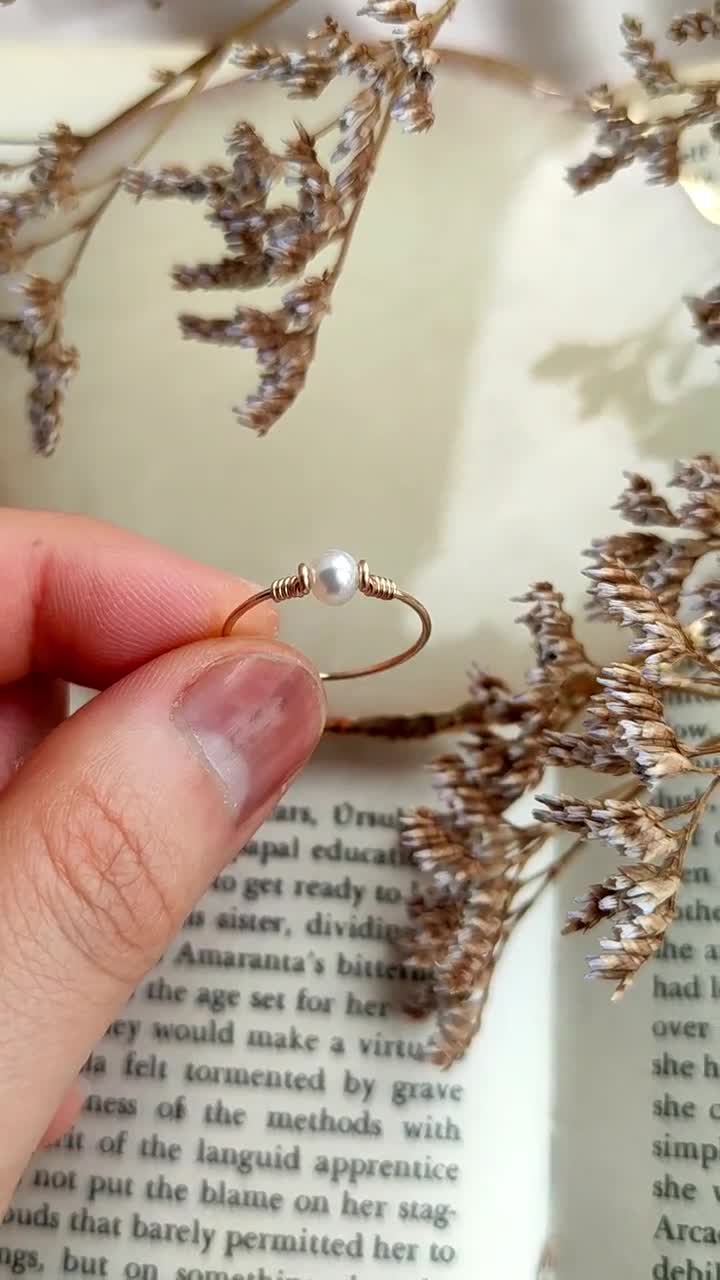In the photograph, a light-skinned hand, possibly belonging to a Caucasian woman, is prominently featured on the left side of the image. Her pinched thumb and index finger are delicately holding a thin, rose-gold ring with a pearl nestled between its bands. Notably, the fingernail on this hand appears bruised, with red and swollen discoloration.

Below and behind the hand, an open book is visible, displaying black printed text, including phrases such as "Amaranta's bitterness" and "they would make a virtue." Part of the text is obscured due to the positioning of the hand. To the right of the hand, dried flowers, possibly baby’s breath, lay across the book’s pages. Adding to the composition, the upper center of the image shows a small, dried brown and blue plant hovering slightly above a beige plate, with intricate leaves displayed prominently. This scene rests upon a white background that further accentuates the delicate details of the objects and the subtle narrative they form.